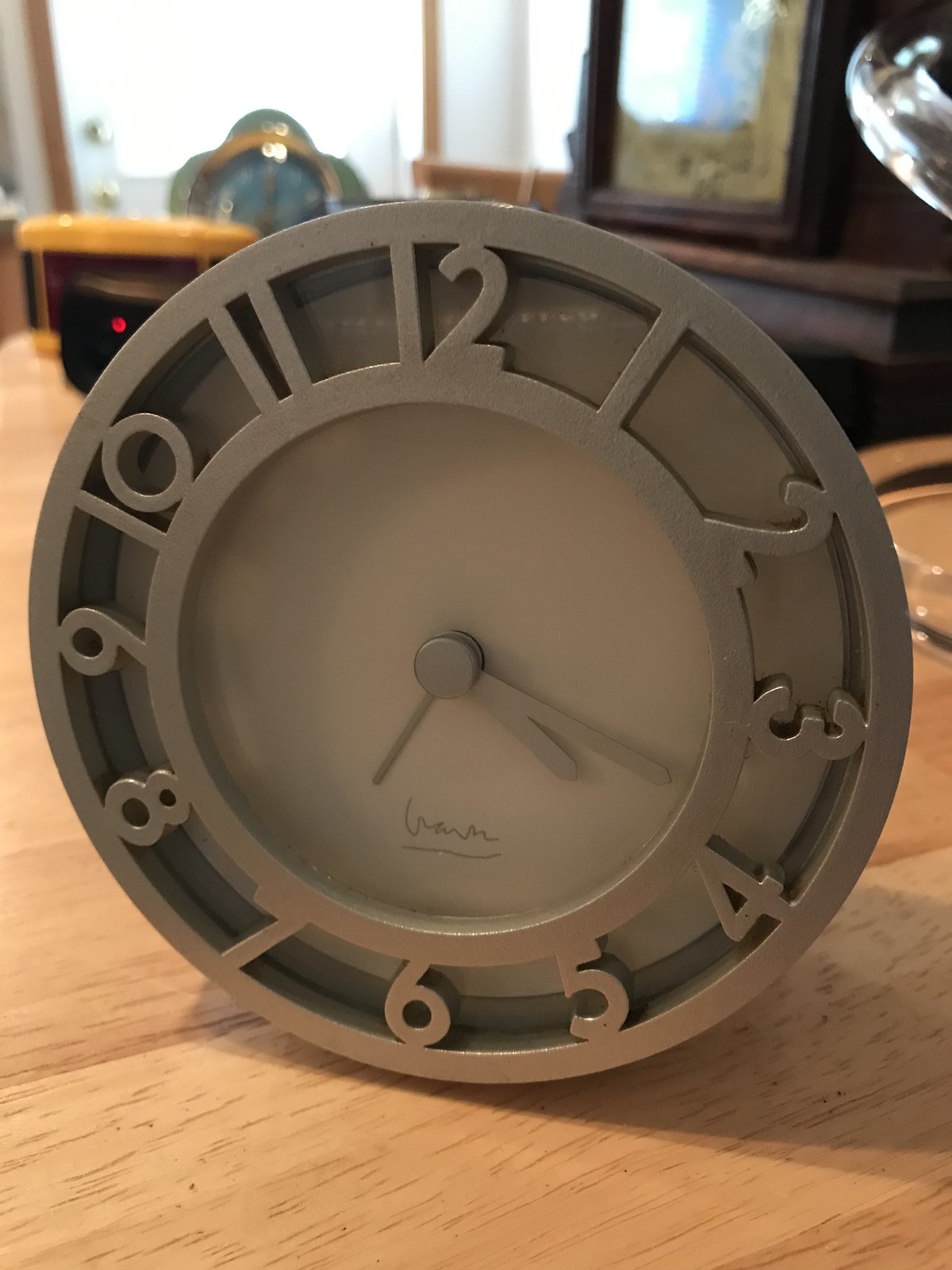A modest, metal clock resembling the rim of a tire sits on a wooden table in a room. The clock features a simple design with numbers 1 through 12 encircling its face. It has three hands: an hour hand, a minute hand, and an additional hand likely indicating an alarm time. The clock displays the current time as approximately 4:18. In the background, an ashtray is visible along with another table further back in the room. This second table has an electronic item on it, identifiable by a small, glowing red light. The room's door and other details of the interior subtly frame the scene, adding depth to the setting.